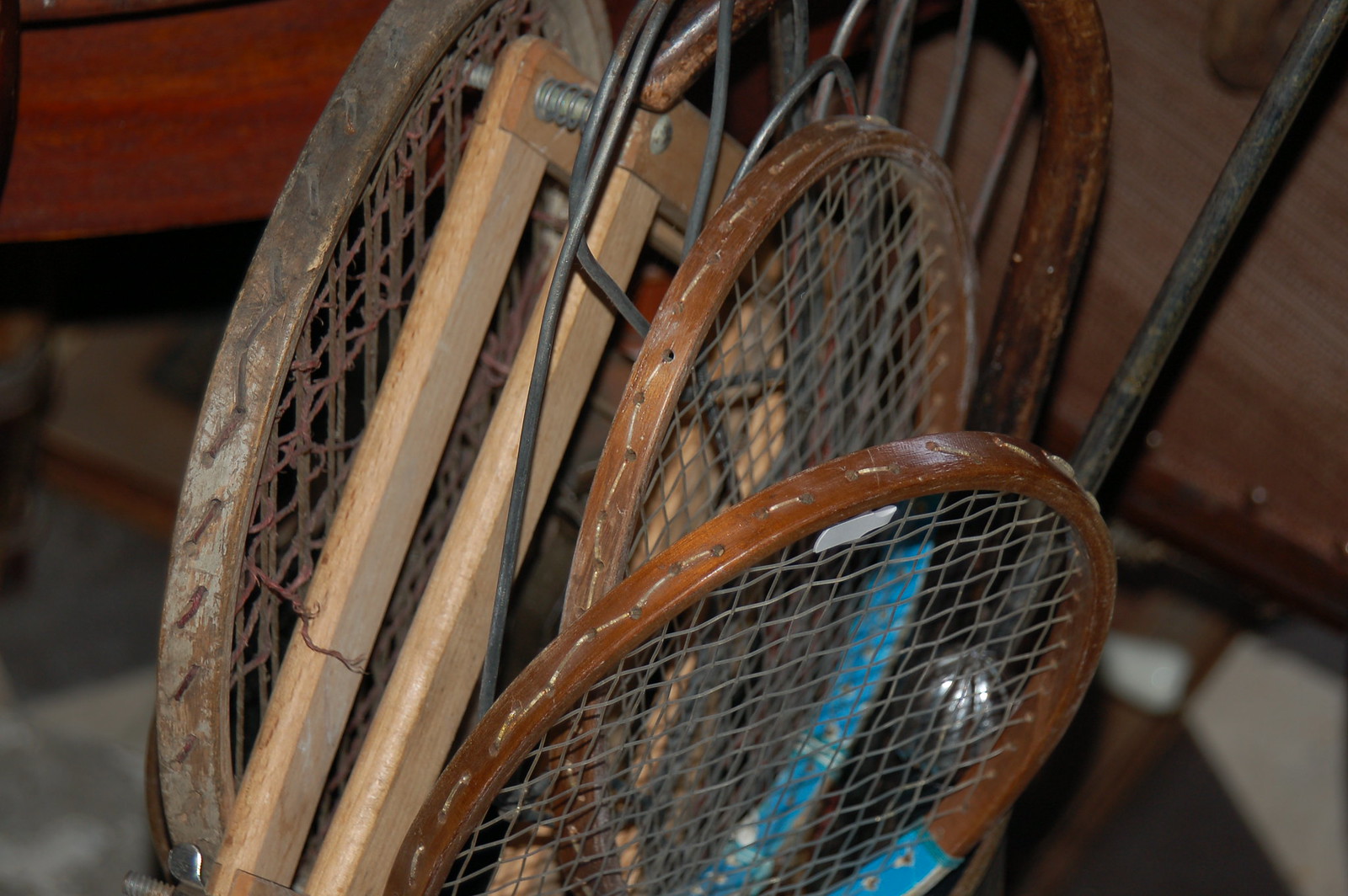The image captures three old, beat-up tennis rackets positioned within a wooden frame, which seems to function as a brace to maintain their shape and prevent bending. The arrangement includes two rackets on the right with brown edges and a gray netting, and one darker racket on the left. The frame is connected by a metal screw at the top left corner. The rackets are filled with their original strings, suggesting they haven't been used in some time. They rest among an assortment of unidentifiable items, which collectively give the impression of a garage sale, used sporting goods store, or pawn shop setting. In the background, there is a mix of dusty, aged objects including a brown wooden chair and a round table, enhancing the nostalgic, cluttered atmosphere.